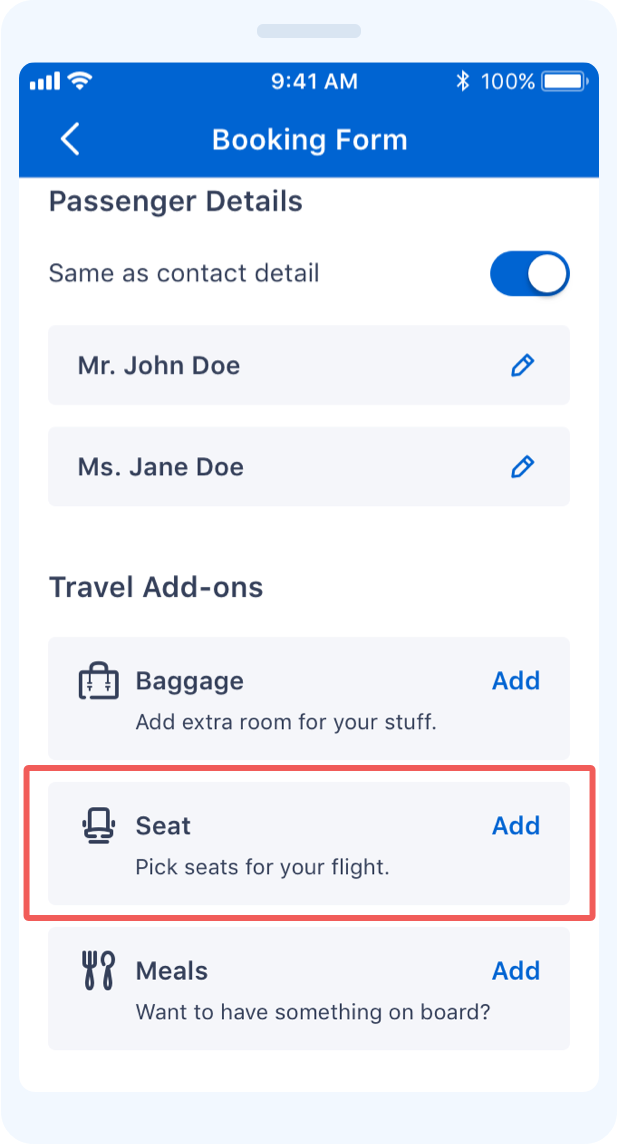This screenshot captures a section of a booking form interface, where the surrounding elements are defined by a thin light blue border. At the top of this border is a gray line. Below this, a darker blue box displays several white icons: a Wi-Fi signal icon, a white arrow, the time "9:41 AM," a "booking form" label, a Bluetooth icon, a 100% battery indicator, and a battery icon with a white indicator. 

Beneath these icons, against a white background, the text in black reads, "Passenger details same as contact detail." A white circle within a blue box appears next to it, followed by two gray boxes, each featuring blue pencil icons and labeled "Mr. John Doe" and "Miss John Doe."

As the form continues, it includes a section titled "Travel Add-Ons." Here, a gray box bears the text "Baggage add extra room for your stuff" alongside a blue luggage icon and an "Add" button in blue.

The next add-on box, outlined with a red-orange border for emphasis, highlights the option to "Pick seats for your flight" in gray text. This section features a blue "Add" button and a seat icon.

The final gray box pertains to meal selection, with the prompt "Meals want to have something on board" and showcases a blue "Add" button accompanied by small fork and spoon icons.